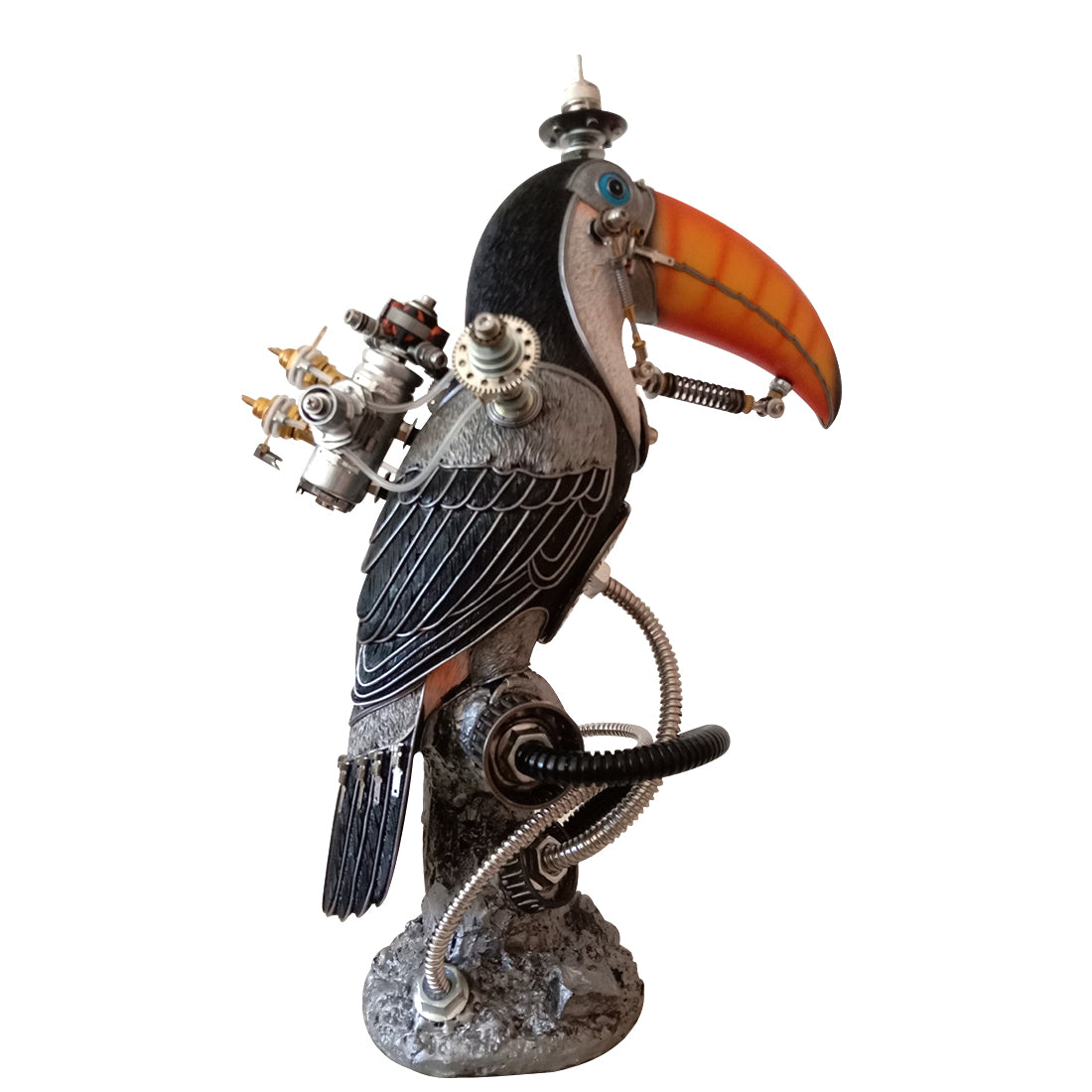This is a photograph of an intricately designed steampunk-style toucan sculpture primarily crafted from metal and glass. The toucan, colored in natural hues with an orange beak featuring concentric red bands, faces to the right. Perched atop a metal, slag-like base, the sculpture boasts a plethora of metal tubing and hoses running in and out of the base and connecting to the toucan’s chest cavity. The bird’s beak is attached to a spring mechanism, allowing for potential movement, highlighted by a bolt drilled into its side. Atop its head is a distinctive candle-like protrusion, resembling a small steel hat or a sewing bobbin. The toucan's large blue eye, detailed with a black metal pupil, contrasts with its white front face and black-painted patches.

The toucan's body is marked by grey wings with black feathers accented by white outlines, and it carries a steampunk-style jetpack-like apparatus on its back. This "jetpack" includes a stainless steel canister, reminiscent of an asthma inhaler, adorned with brass fittings and connected to the tubes surrounding the sculpture. The overall design, composed of various bits of metal and junk, gives the sculpture a whimsical yet mechanical aesthetic, fitting the steampunk genre. Brass elements and pipe fittings add an antique touch to the otherwise gray and black-toned creation.